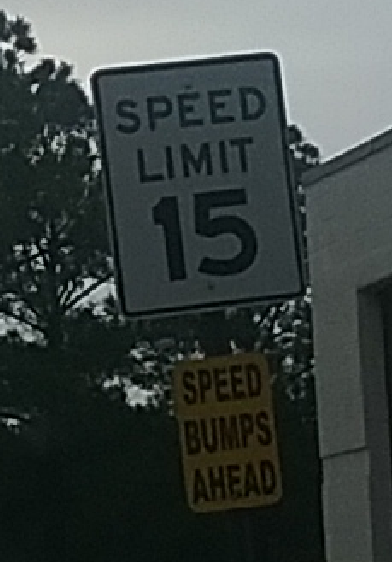This color photograph, taken outdoors just before sunset, showcases a slightly low-resolution image focusing on a street sign. The sky, almost entirely white with barely any blue hues, sets a muted backdrop. Prominently, a speed limit sign indicating "15" in black lettering on a white background stands slightly crooked, pointing to the left. The sign is bordered with black and attached to a post with visible screws. Directly below it, a smaller yellow sign with capitalized red lettering reads "Speed Bumps Ahead."

To the left of the signs is a line of trees with lush foliage, while on the right, part of a concrete building's roof structure is visible, hinting at a possible park-like environment. The lighting is dim, contributing to the hazy, almost grayish appearance of the sky, indicative of dusk.